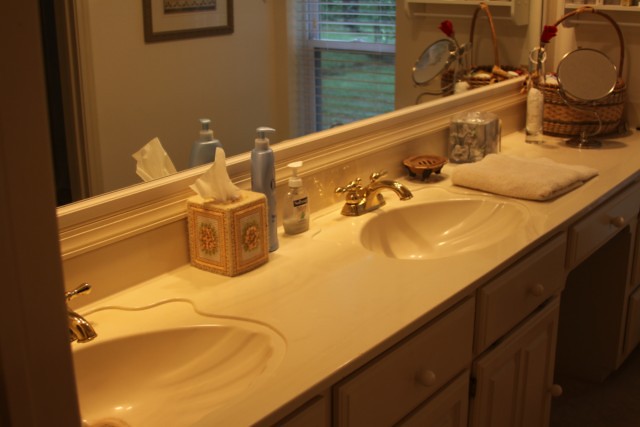The bathroom exudes a retro charm, likely from the 1980s or 1990s, featuring a double sink vanity with seashell-shaped basins and gleaming chrome faucets. The counter and sinks are a unified creamy color, harmonizing with the light, warm-toned wooden cabinets below. Positioned centrally between the two sinks is a floral-patterned tissue box, flanked by a light blue metallic bottle of body lotion with a pump top, and a clear hand wash bottle with a white pump. A soap dish and a neatly folded white towel sit to the right of one sink, accompanied by a basket and a makeup mirror. Above the counter stretches a full-length mirror, reflecting a framed picture on the opposite wall, and an open window revealing green outdoor scenery filtered through mini-blinds.